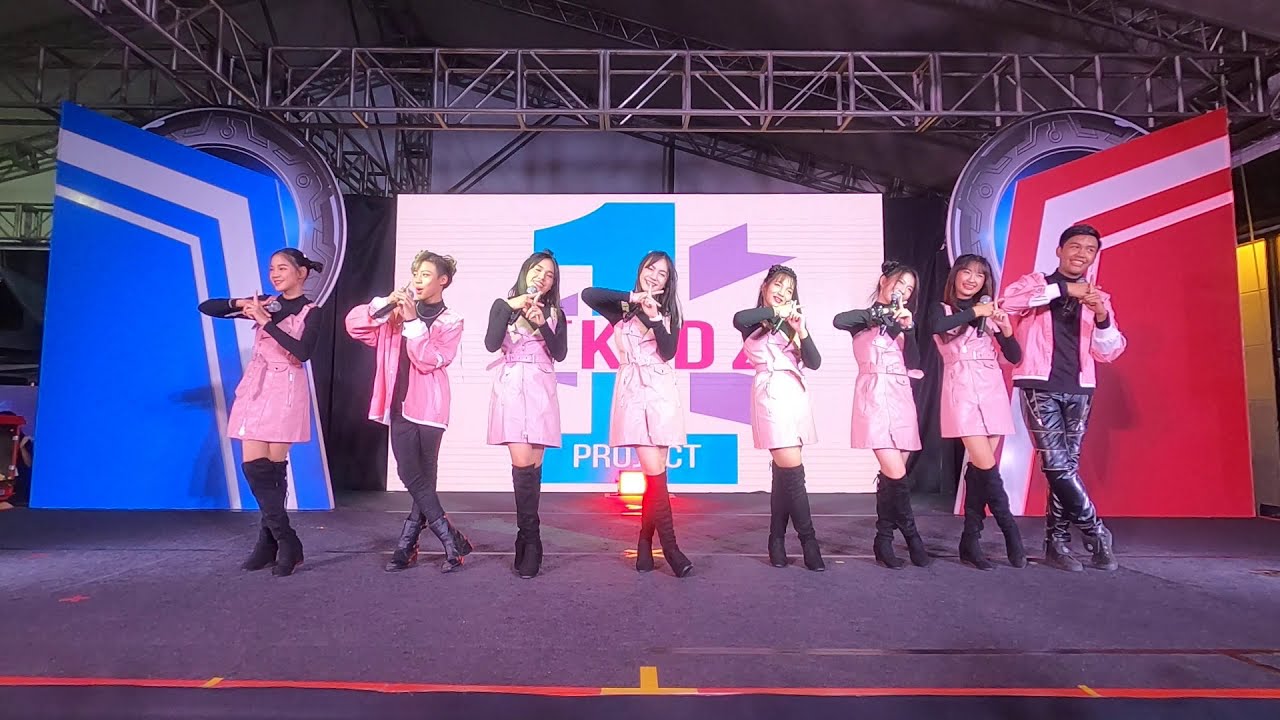The image depicts an indoor performance stage featuring a diverse cast of Asian performers. The stage has a gray floor and is adorned with a variety of colors including red, brown, black, tan, pink, purple, different shades of blue, white, and silver. In the center of the image, seven females and one male are prominently positioned, engaging in expressive hand gestures. The females are clad in pink jackets with dark thigh-high boots, except for one woman who is wearing black pants like the male performer. A large blue structure and bright blue constructs are visible in the background, which also contains intricate metal scaffolding typical of stage settings. Despite the absence of any clearly readable text, there is a display featuring the number one and letters K and D, hinting at possible words like "kid" or "kind." The overall scene suggests an orchestrated performance, enriched with vibrant colors and dynamic expressions.